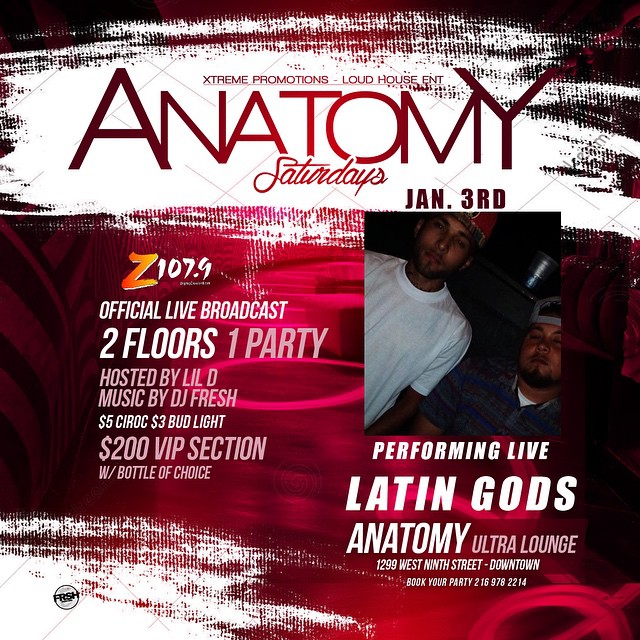This is a promotional flyer for Extreme Promotions' Loud House event at Anatomy Ultra Lounge, set against a striking background of red, white, and black. At the top, bold red text announces "Extreme Promotions, Loud House and Anatomy," with the day "Saturdays" written below in small cursive, and "January 3rd" in black positioned just to the right. Dominating the flyer is a dark image of two men staring directly into the camera, both sporting backwards baseball caps and goatees—one in a white t-shirt and the other in a striped blue and gray t-shirt.

Below their photograph, white text details the main attractions: "Performing Live, Latin Gods." Additional event information follows with the venue name and address: "Anatomy Ultra Lounge, 1299 West 9th Street, Downtown," and a booking contact number: "216-978-2214." To the left of the image, the radio station "Z107.9" is prominently featured in yellow text, noting that they will host an "Official Live Broadcast." The flyer further entices with promises of "Two Floors, One Party," hosted by Lil D and featuring music by DJ Fresh. Drink specials include "$5 Ciroc" and "$3 Bud Light." VIP sections are available for "$200," which includes a bottle of choice. This flyer clearly promotes an exciting night out at Anatomy Ultra Lounge on January 3rd.